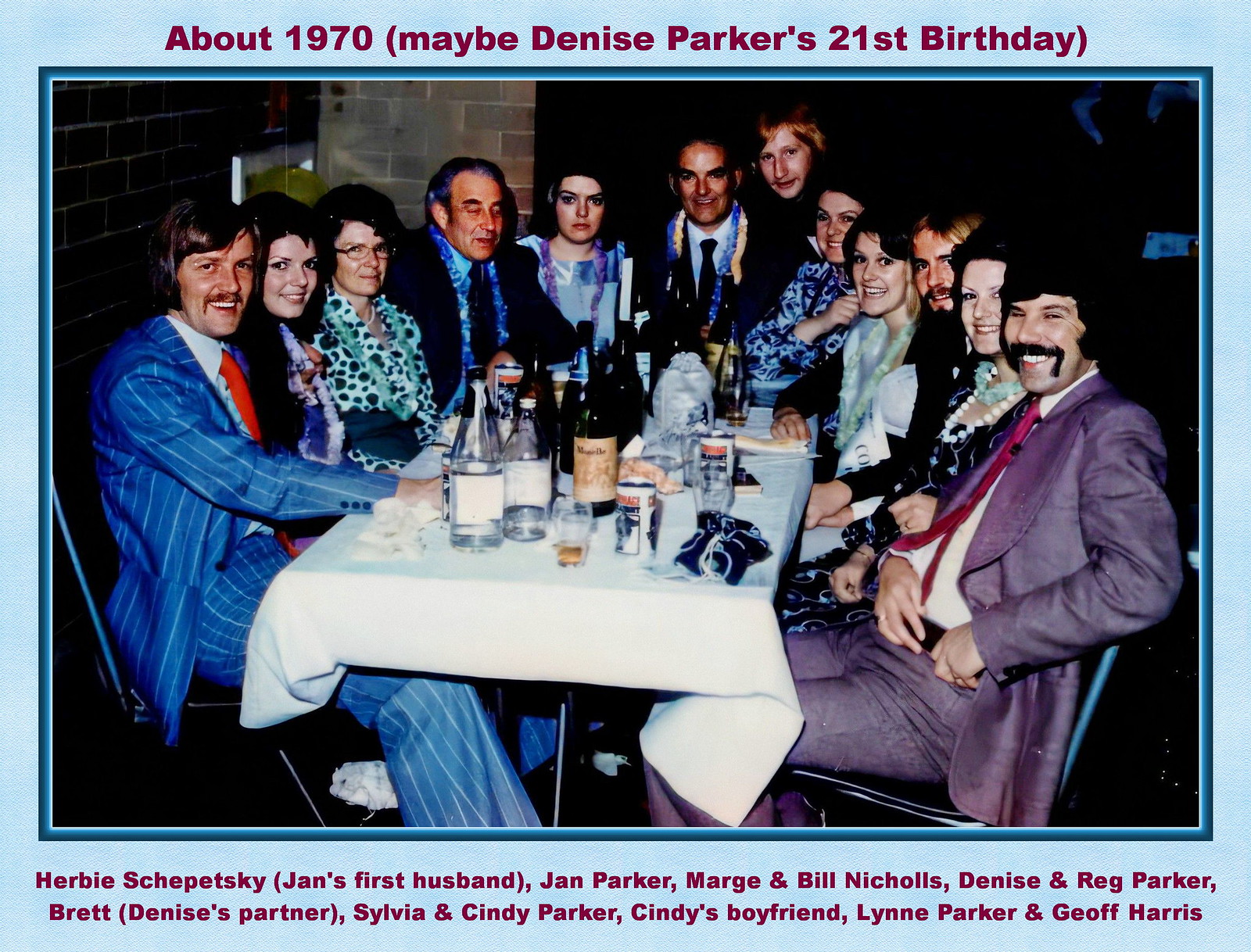This photograph, likely taken in the 1970s, features a large group of 10 to 15 people seated around a rectangular table adorned with a white tablecloth, empty liquor bottles, and glasses. The scene appears old-fashioned, with both men and women dressed in 70s-style outfits, some smiling at the camera while others wear neutral expressions. The image has a blue border, with text at the top in brown or red letters that reads, "about 1970, maybe Denise Parker's 21st birthday." The background reveals brick walls and columns, mostly shadowed. At the bottom of the photograph, names of the individuals are listed: Herbie Shepetsky (Jen's first husband), Jen Parker, Marge and Bill Nicholas, Denise and Greg Parker, Brett (Denise's partner), Sylvia and Cindy Parker, Cindy's boyfriend, Lynn Parker, and Gio Ferris. Notably, two men in the foreground are described: one wears a blue pinstripe suit, and the other a gray suit jacket with gray pants.